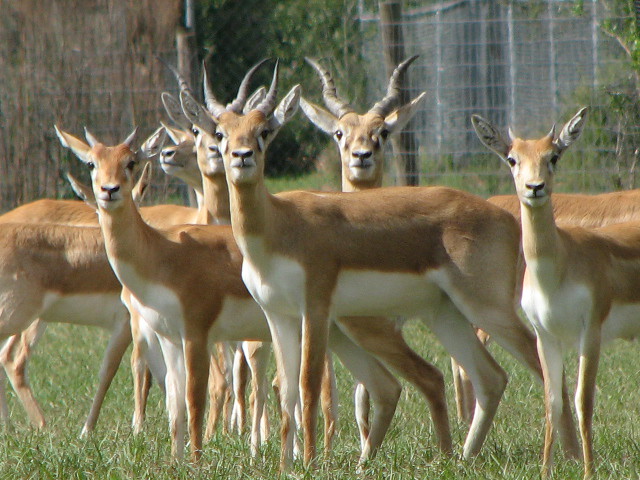This photograph features seven gazelle-like animals standing together in a grassy area with a fence and some brush in the background, indicating they are likely in a preserve or zoo. All seven animals are gazing directly at the camera, creating a captivating and somewhat amusing scene. These creatures have brown fur on their upper bodies and white fur on their chests, bellies, and around their noses and eyes. They sport a variety of horn sizes: the two in the middle have the longest, most curvy horns, while those on the ends have shorter horns, with the smallest one on the far right having notably short horns and prominent ears. They all display a consistent coloration with fawn-colored faces, black noses, mouths, and eyes framed by white fur. Despite some variability in size and horn length, all the animals appear healthy and alert, enjoying a sunny day in their enclosure. The detailed textures of their fur and the vibrant greenery of the grass add to the lively, natural feel of the image.